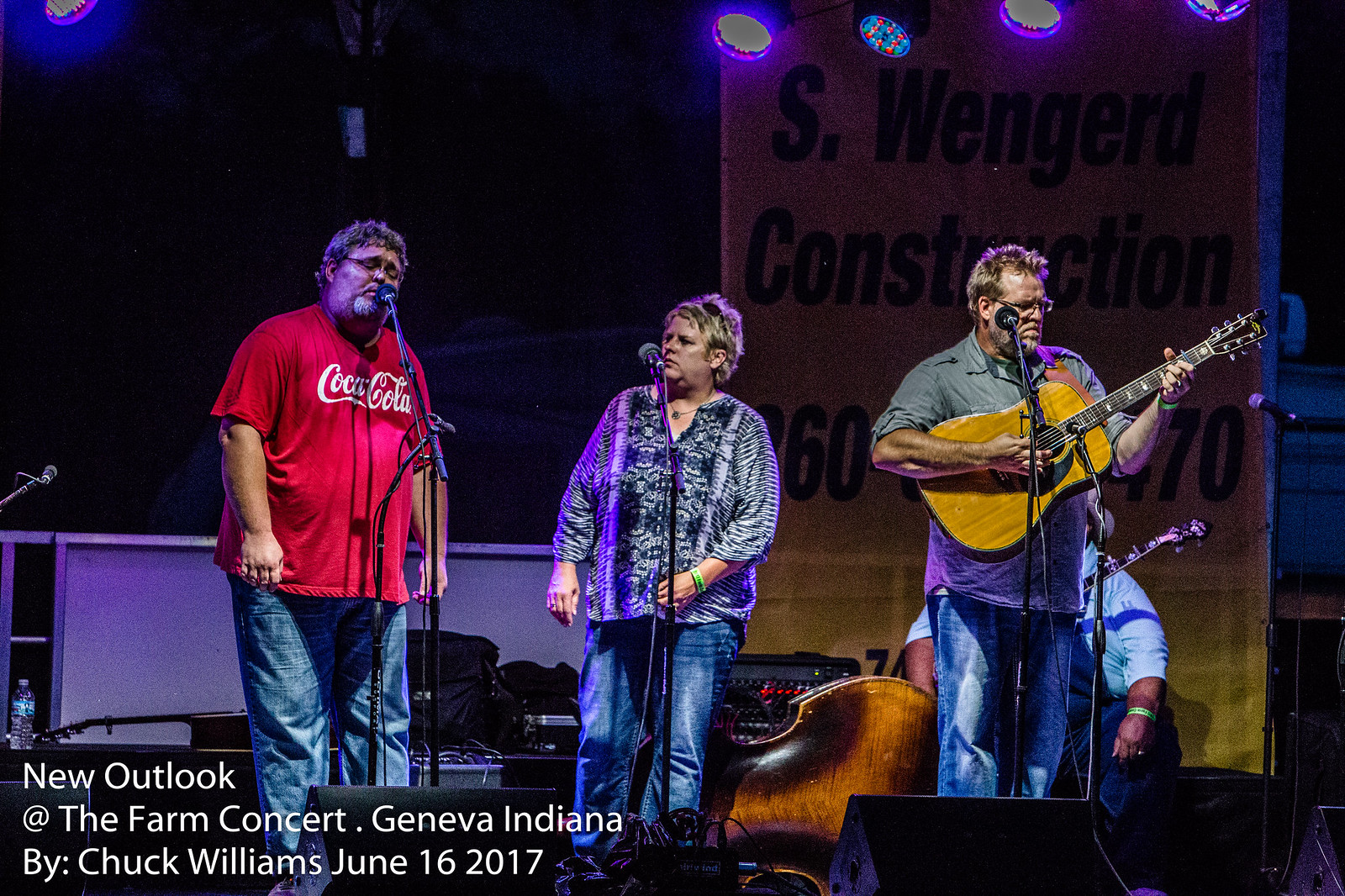The image features three people on a stage, all appearing to be engaged in a musical performance with microphones on stands. From left to right:

- The man on the left is in the middle of singing, wearing a red Coca-Cola t-shirt, blue jeans, and exuding energy into his performance.
- The woman in the center sports a dark blue and light blue blouse with a zigzag design, blue jeans, and a green wristband on her left wrist. She seems to be looking towards the man in the Coca-Cola t-shirt.
- On the right, another man is playing a brown acoustic guitar. He has glasses, sandy blonde hair, a gray button-down shirt, and blue jeans. Behind him, partially obscured, is another person sitting in a chair. 

The stage background includes yellow banners with black lettering that say "Espringer Construction," although the phone number is not visible. Additionally, a bass instrument can be seen on the ground behind the three performers, who all appear comfortable and well-prepared for their act.